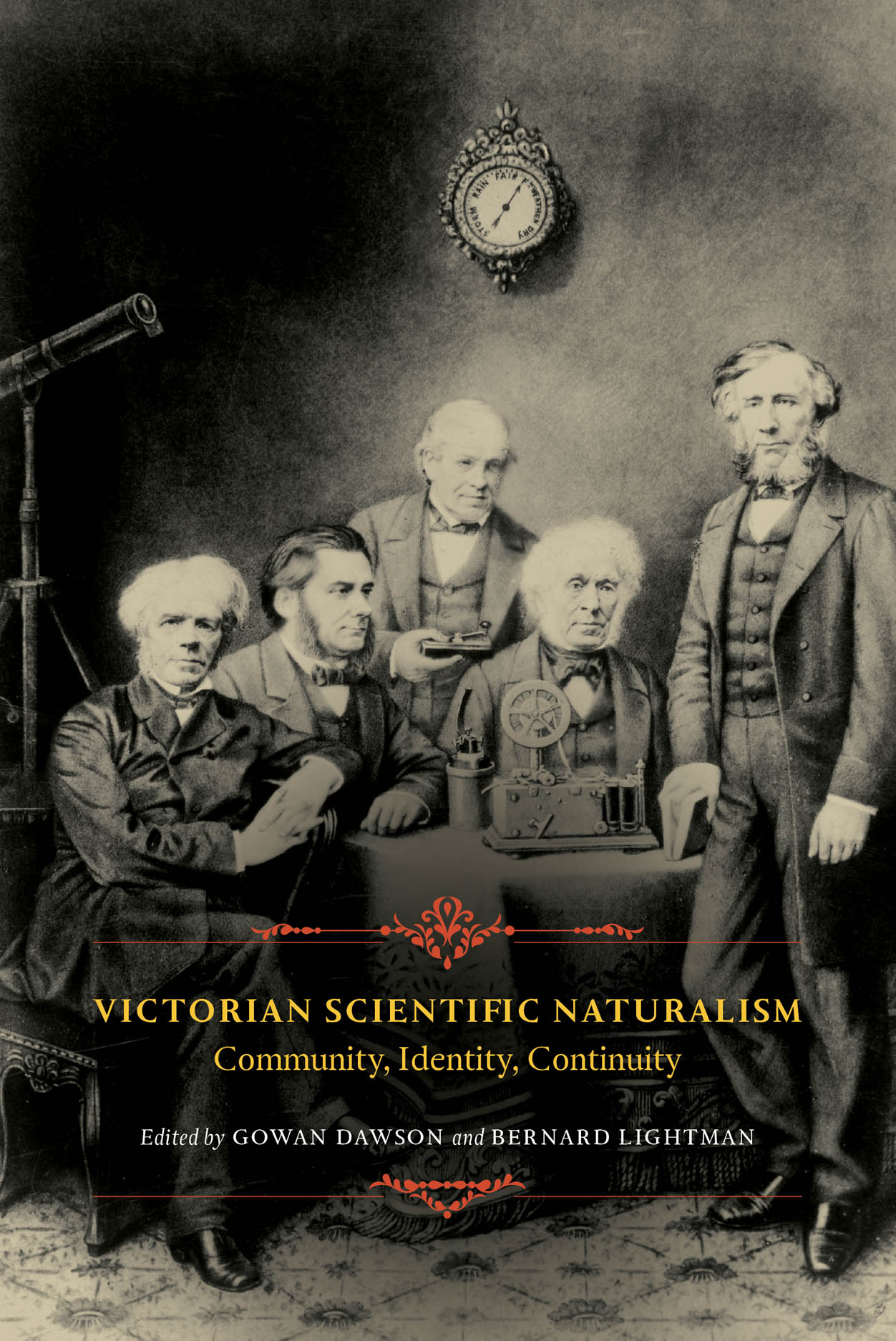The image is the black-and-white cover of a book titled "Victorian Scientific Naturalism: Community, Identity, Continuity," edited by Gowan Dawson and Bernard Lightman. The cover features an old photograph, likely from the late 1800s, showcasing five Caucasian men who appear to be scientists or inventors. These men are arranged around a small table, with three seated and two standing. 

One man stands at the back holding a push-button bell, reminiscent of Pavlovian experiments. The second man from the left, seated, has dark hair, while the others have graying hair. All five are dressed in formal attire, including knee-length jackets, suits, and some bow ties. The men are engaged with a few unspecified mechanical items on the table, possibly scientific instruments, adding to the scholarly atmosphere.

In the background, a clock hangs on the wall, and a telescope is positioned to the left of the group. The setting exudes a sense of historical scientific inquiry. The title text is prominently displayed in large yellow lettering at the bottom of the cover, with the editors' names in white below it. Decorative floral designs with red accents frame this text, adding an ornate touch to the otherwise monochromatic theme. The overall scene and attire emphasize the scholarly and historical context, characteristic of Victorian scientific endeavors.